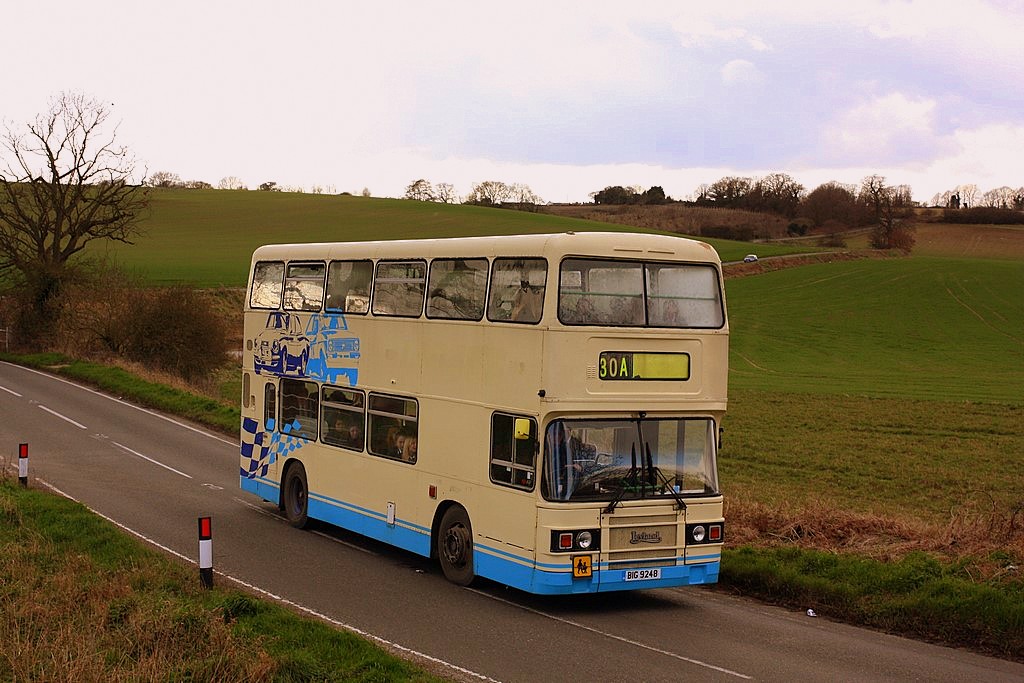The image depicts a beige double-decker bus driving on a two-lane, one-way country road, surrounded by vast fields of green grass and a few leafless trees dotting the horizon to the left. The bus, adorned with a thin blue ribbon around its base and additional blue paint illustrating two cars, features a black text reading "30A" on a yellow bar at the top. Although the road appears very narrow and reminiscent of pre-1970s construction, it is well-marked with white lines. The sky is cloudy, contributing to the serene rural atmosphere. Despite the bus's motion seeming indeterminate, there are visible passengers on both the lower and upper decks, adding life to the tranquil countryside scene.